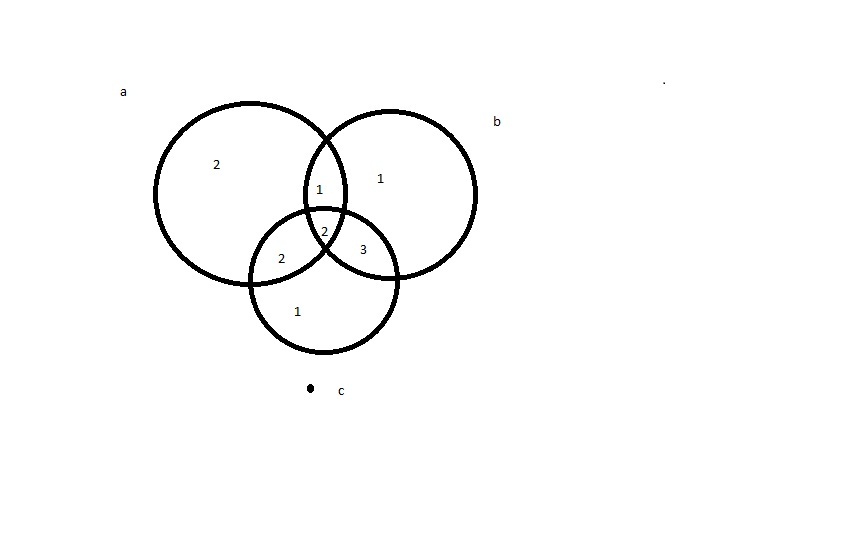This computer-generated image features three circles of varying sizes in a partially overlapping arrangement. The left-most circle is marginally larger than the one on the right, and these two circles intersect to create a hoop effect. Below them is a smaller circle that also overlaps with the other two. Collectively, these circles converge towards the center of the image.

Each circle is annotated with specific letters and numbers. The larger left circle has a lowercase 'a' positioned outside its upper left perimeter and contains the number '2' within its boundary. The area where this circle intersects with the right circle displays the number '1', indicating shared space.

In the central overlapping region where all three circles converge, there are two instances of the number '2', a '3' within the right circle, and a '1' in the lower circle. The right circle itself includes an internal '1' and has a lowercase 'b' positioned outside its boundary. Similarly, the lower circle features a lowercase 'c' with a dot right outside its border.

Altogether, the visual arrangement and annotations create a complex and detailed geometric composition.